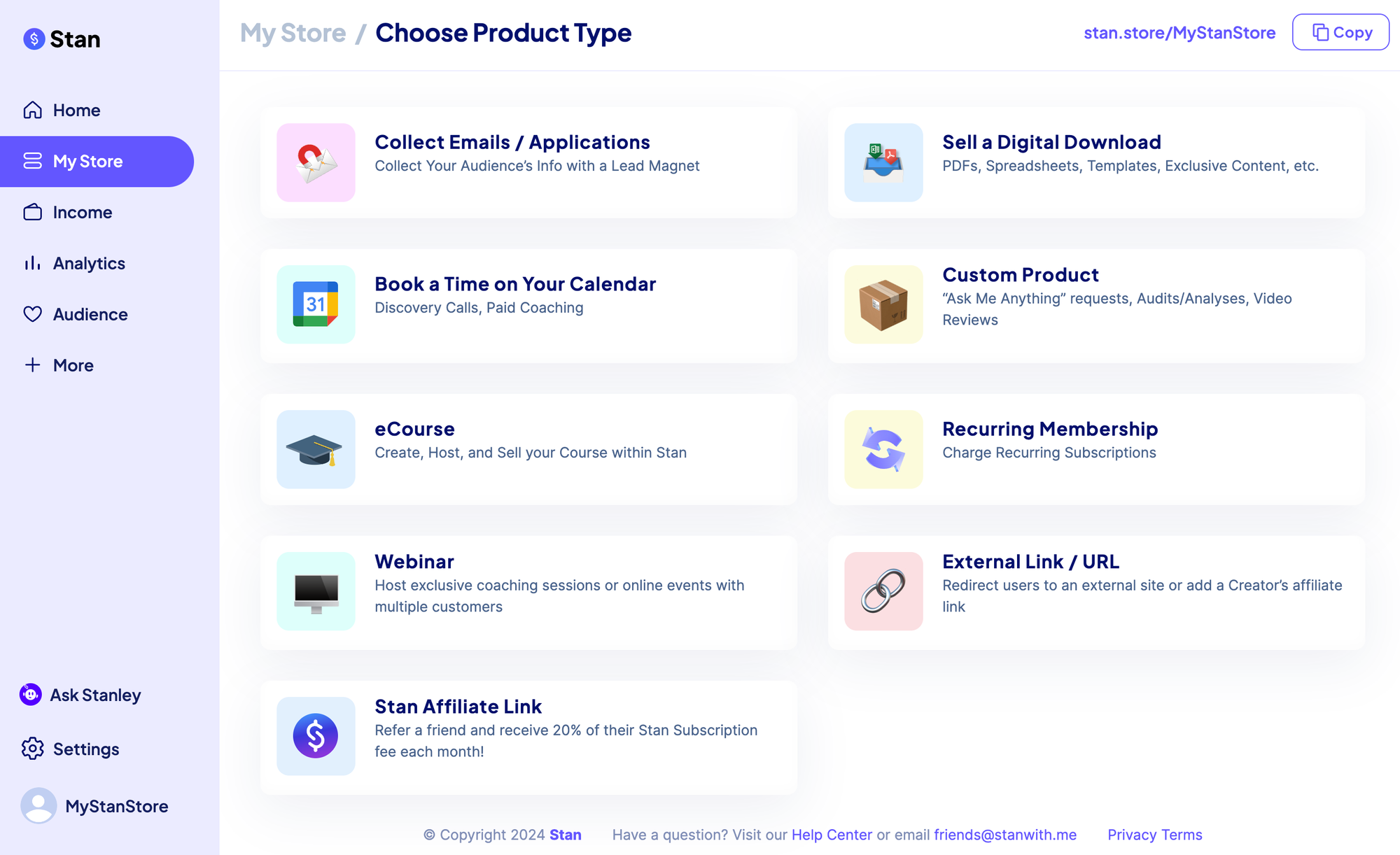The image appears to be a screenshot from a website with navigation and various product options. On the left side, there is a blue vertical navigation bar featuring categories such as "Stan," "Home," "My Store" (highlighted in blue), "Income Analytics," "Audience," "More," "Ask Stan," "Lease Settings," and "My Stan Store."

At the top, "My Store" and "Choose Product Type" are prominently displayed. On the right, there is a section titled "My Stan's Store," which includes a grid of icons arranged in rows, each representing different options available in the store. Here's a detailed breakdown of each icon and its description:

1. **Collect Emails**:
   - Description: Applications, Collect Your Audience's Info with a Lead Magnet.
   - Icon: Represents a lead magnet.

2. **Sell Digital Downloads**:
   - Description: PDFs, spreadsheets, templates, exclusive content, etc.
   - Icon: Diverse file icons, including a blue word icon and a spreadsheet icon.

3. **Book Time on Your Calendar**:
   - Description: Scheduling appointments.
   - Icon: Calendar date showing "31."

4. **Custom Product**:
   - Description: Various personalized products.
   - Icon: Brown box.

5. **Ask Me Anything Requests**:
   - Description: Audits, Analysis, Video Reviews.
   - Icon: Unspecified.

6. **eCourse**:
   - Description: Create, Host, and Sell Your Course with Stan.
   - Icon: Blue mortarboard (graduation cap).

7. **Recurring Memberships**:
   - Description: Charge Recurring Subscriptions.
   - Icon: Two blue reload arrows.

8. **Webinar**:
   - Description: Host Exclusive Coaching Sessions or Online Events with Multiple Customers.
   - Icon: Computer screen against a blue background.

9. **External Link URL**:
   - Description: Redirect users to an external site or add a creator’s affiliate link.
   - Icon: Two interlocked chain links against a pink background.

10. **Stan Affiliate Link**:
    - Description: Refer a friend and receive 20% of their Stan subscription fee each month.
    - Icon: Dollar sign in a blue circle against a light blue background.

At the bottom of the webpage, there is copyright information.

This caption should give viewers a comprehensive and detailed understanding of the various elements and functionalities displayed in the screenshot.